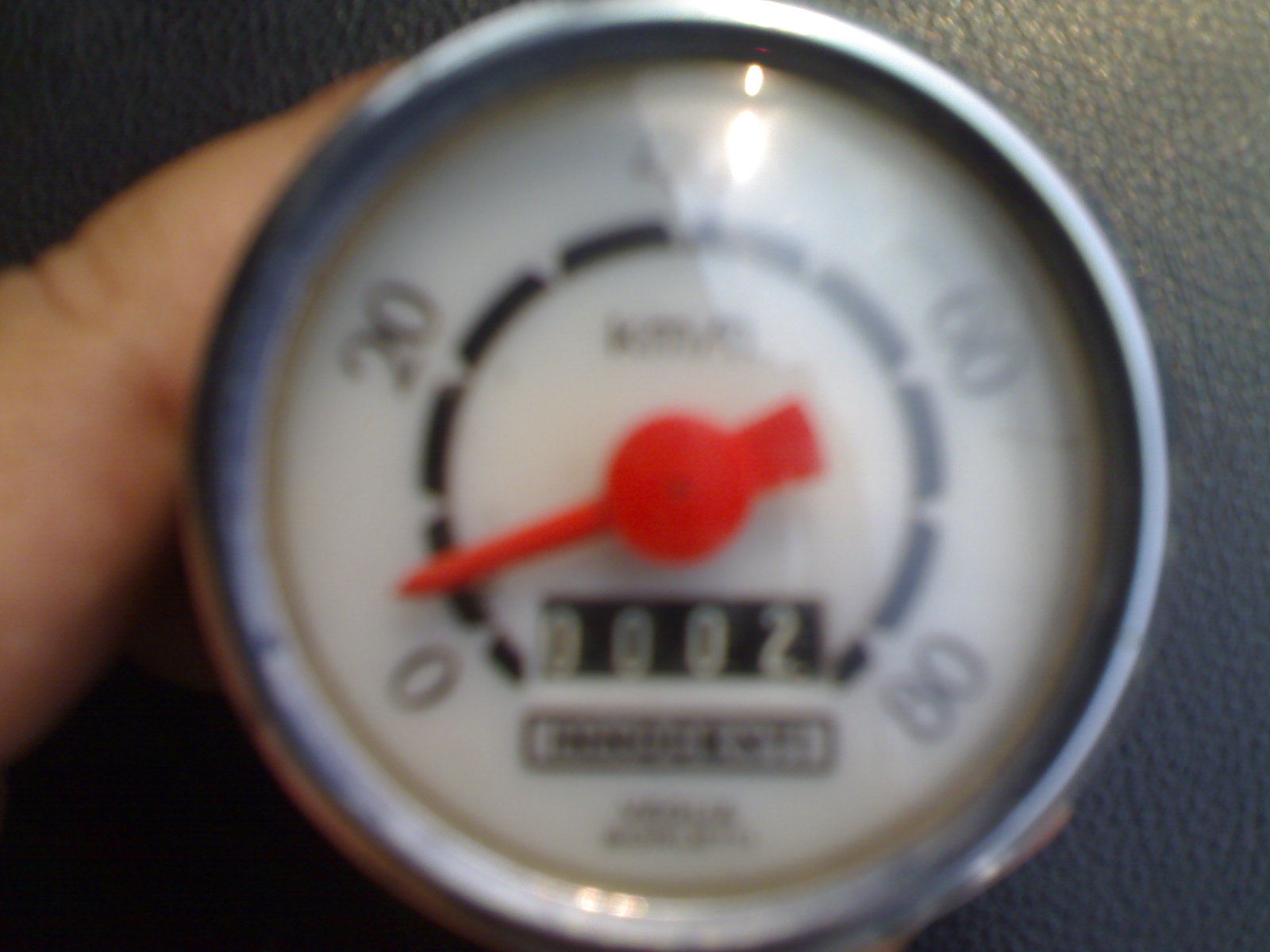The image depicts a severely out-of-focus pedometer or speedometer, which seems to be designed for measuring speed, possibly on a bike. The device features a central dial with a hand pointer that indicates the speed. The pointer, characterized by a long, thin needle extending from a rounded center with a dark spot, is currently indicating a speed of around 5 units, though the exact measurement is unclear because the photo is out of focus. The surrounding rim of the device is shiny metal, giving it a polished appearance.

Just below the pointer, the numbers "002" are visible, suggesting that the device has recorded a very minimal distance or speed. Further below, a black rectangular section with unreadable lettering is present, followed by more black text that is also indistinct. The speedometer dial includes clearly visible numbers marking speeds: 0, 20, 40, 60, and 80. The number 40 is particularly highlighted by a light, aiding in its identification despite the blurriness.

The device is held by someone, with only one finger prominently visible holding it. The background consists of a dark grey, dappled surface that contrasts with the chrome detailing of the speedometer, making it stand out more. A small patch of brown is visible to the far left, potentially from light reflection, indicating the presence of additional materials or items in the periphery. Despite the overall poor focus, the key structural elements and measurements of the speedometer can be discerned.